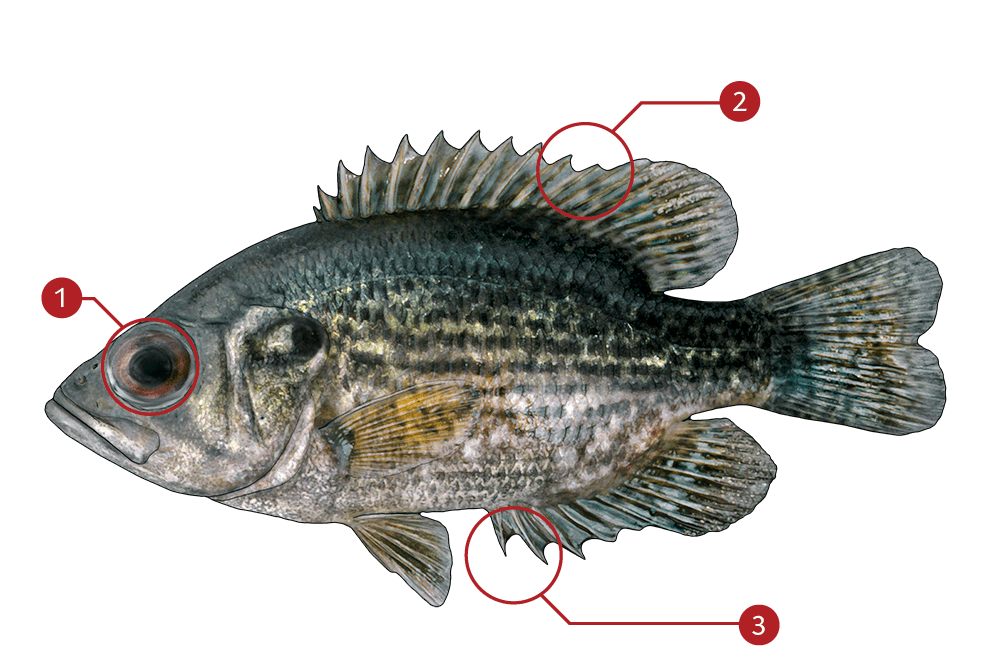This realistic rendering of an oval-shaped fish captures its complete side profile, displayed isolated on a white background. The fish faces left, showcasing its silvery head and a body adorned with light silver and dark gray scales. Its dorsal area is highlighted with rippled dorsal fins, while its back scales display shades of gray and teal blue. Underneath, the fish features light gray and white scales, with a fan-shaped tail and similar fin structures present beneath its body. The fish's open black eye is distinctly visible. The image includes three red call-out circles with corresponding arrows pointing to particular parts of the fish: number one encircles the eye, number two highlights the dorsal fin, and number three marks the fin at the bottom of the fish's body. The fish's overall shape resembles a spade or clover, akin to card suits.